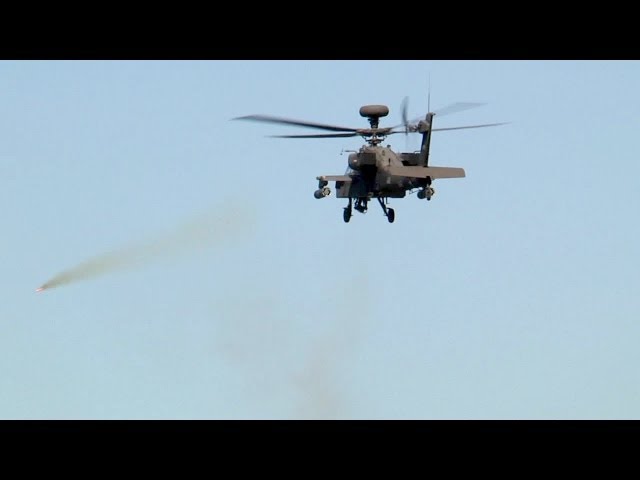The image, framed by thick black borders at the top and bottom, features a scene set against a light blue sky with a slight white haze. Dominating the scene toward the upper right of the center is a gray military-style helicopter facing slightly left. The helicopter, equipped with top propellers and a disc-like structure above them, has distinctive gray wings with mounted guns and a gray back wing with a rudder. Its landing gear consists of two front wheels that are visibly down. On the far left of the image, a fired missile or rocket trails behind the helicopter. The missile, red at its base, emits a plume of dark gray smoke that transitions to a lighter gray and appears to incorporate brown dust as it moves upward and away from the helicopter.